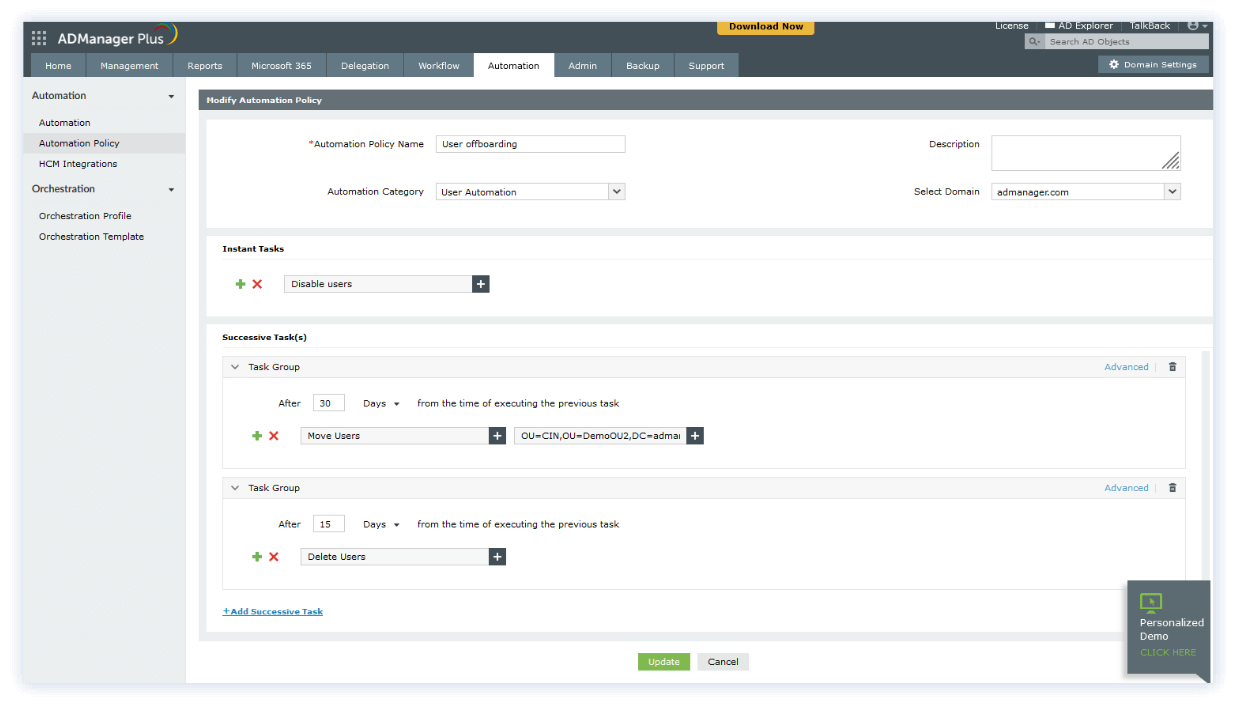Screen capture of an IT management platform titled AD Manager Plus, showcasing a detailed interface focused on automation policy configuration. The interface features a navigation ribbon at the top with multiple tabs including Home, Management, Reports, Microsoft 365, Designation Workflow, Automation, Admin, Backup, and Support.

At the center of the screen, the title "Modify Automation Policy" is displayed prominently. The main page is divided into several sections with input fields and options:

1. **Top Left Section**:
   - **Automation Policy Name**: An input field for specifying the name of the automation policy.
   - **Automation Category**: A dropdown or input field to categorize the automation policy.

2. **Top Right Section**:
   - **Description**: A field to provide a detailed description of the automation policy.
   - **Select Domain**: An option to choose the relevant domain for executing the policy.

3. **Middle Section**:
   - **Instant Tasks**: A section that includes a window labeled "Disable Users," indicating immediate tasks to be performed.

4. **Successive Tasks**:
   - **Task Group**: 
     - First Task Group: Executes a task "Move Users" 30 days after the previous task, with domain-related information provided to the right.
     - Second Task Group: Executes a task "Delete Users" 15 days after the previous task.

This interface clearly outlines the structured process of configuring automation policies, including immediate actions and scheduled tasks with specific time frames for execution, essential for effective IT management.